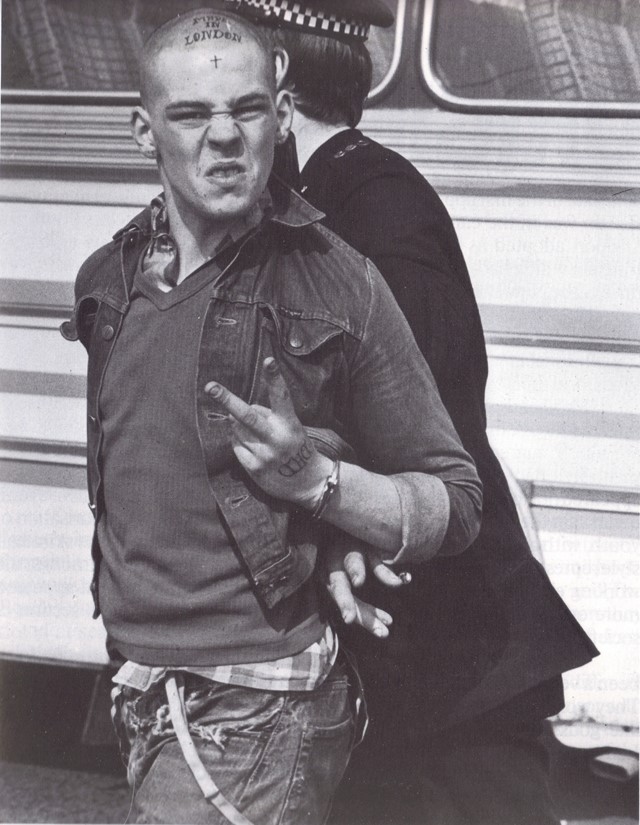In this black-and-white historical photograph, likely from the 1960s or 70s, we see a dramatic scene in front of an old-fashioned bus with distinctive stripes and rounded windows. Dominating two-thirds of the image are two figures: a police officer and a young man, possibly in his teens or early 20s, who appears to be under arrest. The officer, visible only from the side and dressed in a black uniform with a hat featuring a black-and-white checkered band, firmly grips the young man's arm. The young man faces the camera directly, his fair-skinned face contorted in a disgruntled expression, wrinkling his nose and possibly ready to spit. He is outfitted in a jean jacket layered over a dark sweater, with a flannel shirt peeking out from underneath and worn, ripped jeans. Thin suspenders dangle at his sides, and his look is completed with tattoos or crude pen drawings. Prominently, his mostly shaved head features the text "Made in London" with a small cross underneath. He displays a peace sign with his hand, which also bears an unreadable tattoo or scribble. The handcuffs restraining his arm highlight his defiance and complexity, making for a striking and evocative image.